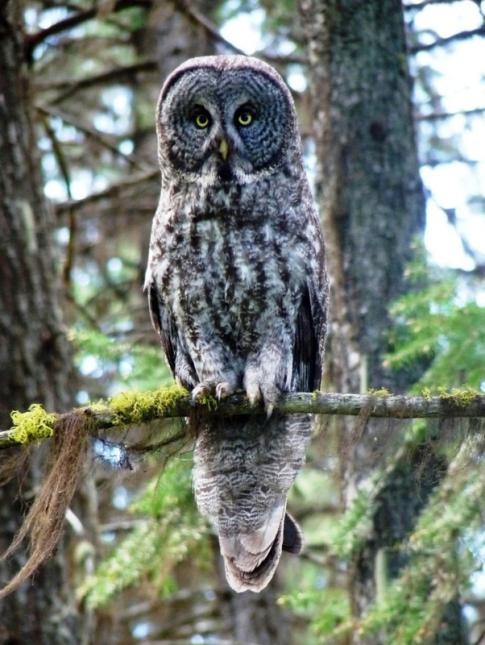In this vivid photograph, a large, gray owl with intricate brown and white flecks is perched on a tree branch in the middle of a dense forest. The owl stands out with its intense yellow eyes, staring directly at the camera, creating a mesmerizing focal point. The branch it perches on, covered in moss, stretches horizontally across the lower third of the image, with the owl’s tail hanging down on the other side. The background reveals an array of trees, some adorned with leaves and others with moss, capturing the depth and lushness of the forest environment. Light filters softly through the foliage, indicating it’s daytime, and adding a serene ambiance to the scene. The owl appears calm yet vigilant, its wings relaxed by its sides, and its feathers ruffled slightly, accentuating its alertness and the fine detail in its plumage. The photograph, taller than it is wide, beautifully captures not only the striking presence of the owl but also the rich, natural intricacies of its woodland habitat.